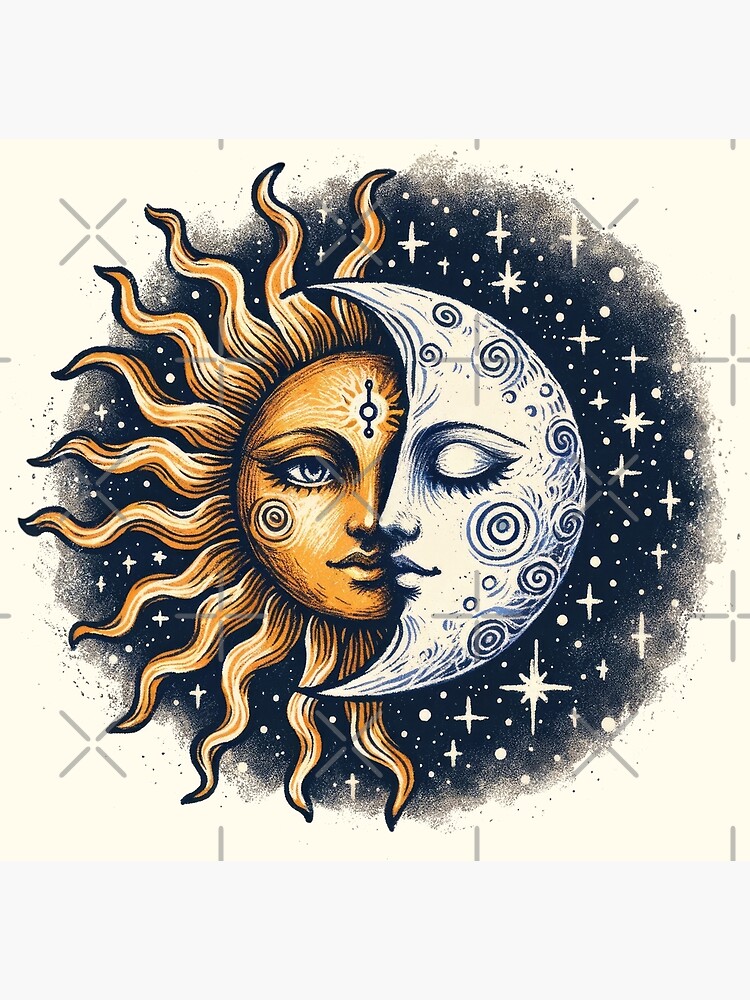This image is an intricate artistic rendering of the sun and moon side-by-side, with both celestial bodies depicted as female faces. On the left, the sun features an open eye, a visible nose, and lips, while its other eye, half of the nose, and lips are concealed by the moon on the right. The sun has long, squiggly rays extending outward, resembling hair, and it is adorned with several symbols on its face. It is depicted in deep orange with white lines running through it. The moon on the right is a crescent shape facing left, with closed eyes and long, lush eyelashes, a defined nose, and lips. The moon is white with black squiggly lines on its surface and has pointed ends at the top and bottom. Behind the sun and moon is a galaxy filled with numerous stars that shine against a blackish-blue background. The overall background is light-colored, surrounding a central black circle that fades into a more tan hue towards the edges. Gray X's in straight lines also surround the central image.